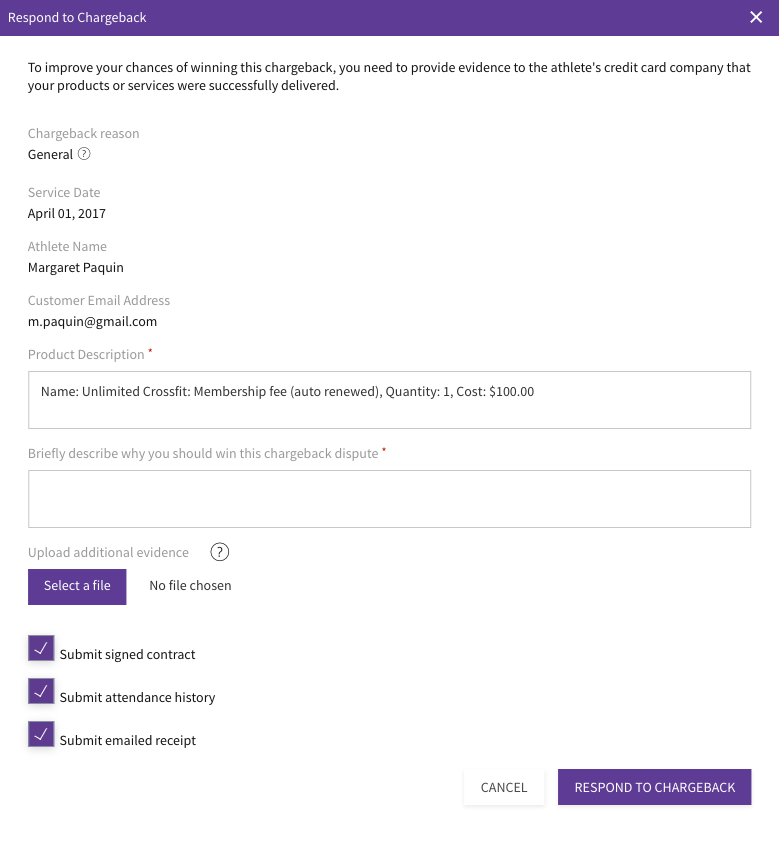The screenshot depicts an online form designed for responding to a chargeback dispute on a financial transaction. At the top left corner, the form is titled "Respond to Chargeback." Below this, the text suggests that to improve the chances of winning the chargeback, the user needs to provide evidence to the complainant's credit card company that the products or services were successfully delivered.

The primary section of the form displays the following details:
- **Chargeback Reason**: General
- **Service Date**: April 1st, 2017
- **Athlete Name**: Margaret Paquin
- **Customer Email Address**: m.paquin@gmail.com
- **Product Description**: 
  - **Name**: Ultimate Unlimited CrossFit Membership
  - **Fee**: $100
  - **Quantity**: 1 unit 

Next, the form asks the user to **"Briefly Describe Why You Should Win This Chargeback Dispute"**, but this text box remains empty in the screenshot.

Subsequently, the form prompts the user to **"Upload Additional Evidence"** with an option to select a file, currently showing "No file chosen."

Below this, three checkboxes are marked, indicating that the following pieces of evidence should be submitted:
1. Submit signed contract
2. Submit attendance history
3. Submit emailed receipt